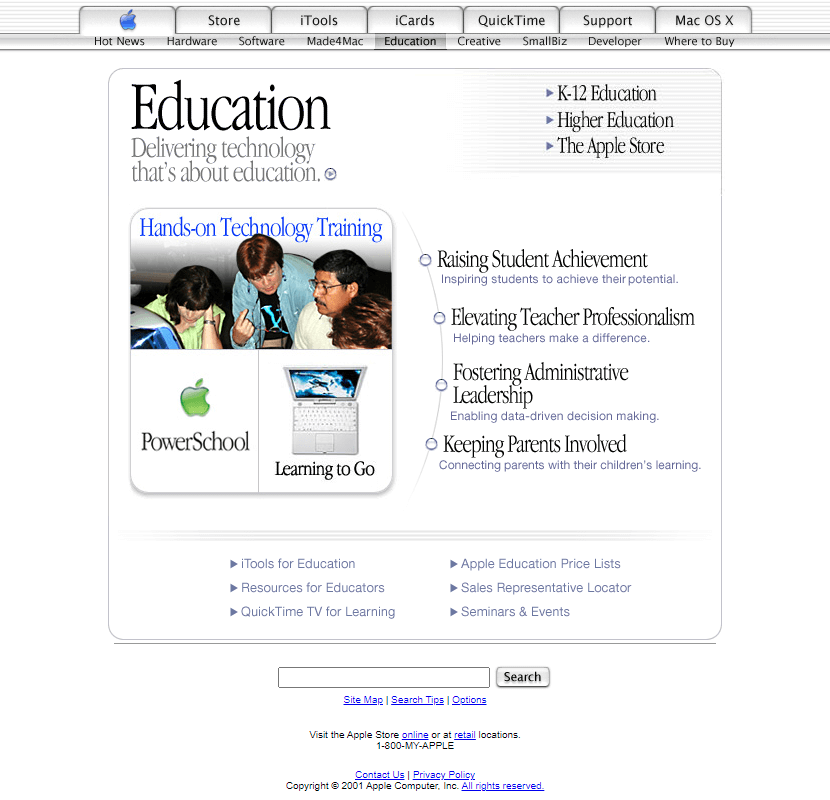The image appears to be a screenshot captured from a computer screen, presented in a vertical format. The background of the image is predominantly white, presumably the default white background of the computer screen. 

At the top of the screen, there is a gray menu bar featuring various tab options, including "Apple," "Blue Apple Tab," "Storm," "iTunes," "iCards," "QuickTime," "Support," and "Mac OS X." Hovering over the "Apple" menu reveals additional dropdown options such as "Hot News," "Hardware," "Software," "Made for Mac," "Education," "Creative," "Small Biz," "Developer," and "Where to Buy."

Centrally located against the white backdrop is a thin, rounded-edge rectangular box. In the upper left corner of this box, there is bold black text that reads "Education," followed by slightly less bold text stating "Delivering Technology That's About Education." On the right side within this box are three clickable options indicated by small arrows: "K-12 Education," "Higher Education," and "Apple Store."

Below these headings, another rounded rectangular section in blue text reads "Hands-On Technology Training." Accompanied within this section is an image featuring four individuals examining an older style Apple computer, all appearing engaged and focused on the screen. 

This section highlights several initiatives including "Power School," "Learning to Go," and portrays a laptop. It also lists educational objectives such as "Raising Student Achievement," "Elevating Teacher Professionalism," "Fostering Administrative Leadership," and "Keeping Parents Involved," each followed by brief explanatory lines.

Towards the bottom of the image, there are various clickable links and tips for additional information. At the very bottom, there is a search bar along with copyright and contact information.

Overall, the image is a detailed and comprehensive representation of an educational technology promotional content from Apple, emphasizing their commitment to supporting education through innovative technology solutions.